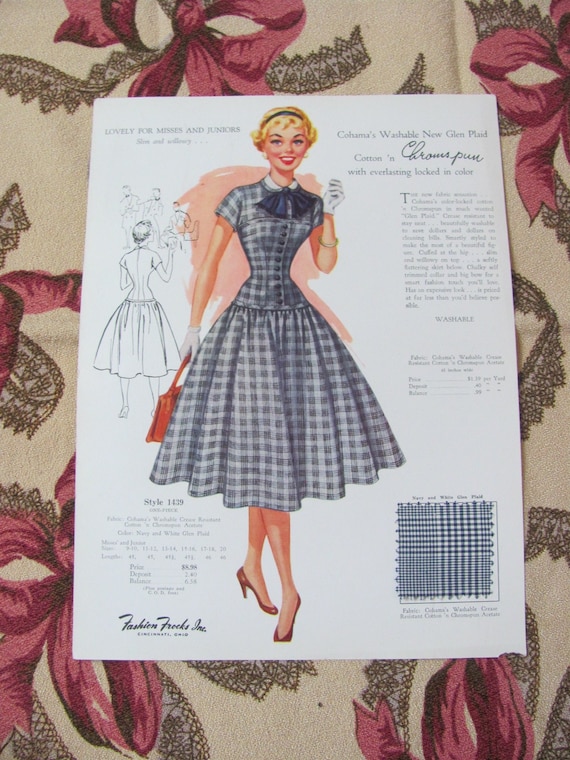This image depicts a vintage sewing pattern cover, likely from the 1940s, designed to create a dress. The cover itself is a white rectangle featuring multiple lines of black text. In the top left corner, it reads, "Lovely for Missus and Juniors," highlighting its versatile appeal. The text details the fabric as "Kahoma's washable new Glenn plaid cotton and cross plum with everlasting locked-in color," emphasizing the durability and quality of the material. 

Central to the cover is a detailed sketch of a woman wearing a stylish, blue and gray checkered plaid dress, complete with black buttons down the top half. She is accessorized with a black headband, gold bracelet, two white gloves, a red purse, and matching red heels. The woman has blonde hair, and beside her is a close-up picture of the plaid print, giving a better view of the fabric's design. To the left of this sketched woman is another sketched depiction showing the back of the dress, providing a comprehensive view of its design.

In the bottom left corner, the text "Fashion Prex Inc" can be seen, while a black and white barcode appears on the right side. The term "washable" is also prominently featured on the right side of the image. The cover is set against a tan table adorned with a crown-like design and pink ribbons, adding to the vintage aesthetic. The overall layout and detailed illustrations suggest that this is a pattern packet, similar to those produced by brands like McCall, intended for home sewing enthusiasts.